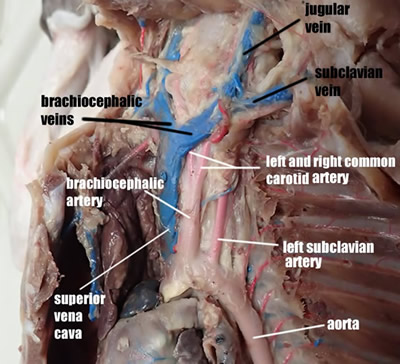This image is a detailed medical illustration, possibly a cadaver dissection, showing a realistic and labeled view of the human thoracic and neck region. The image features prominently colored veins and arteries, such as the blue jugular veins and subclavian veins, as well as the pink brachiocephalic veins. It also includes the brachiocephalic artery, aorta, superior vena cava, left and right common carotid arteries, and the left subclavian artery, with the text labels in blue and white identifying these anatomical structures. The heart and sections of the rib cage are visible, suggesting a close-up view that highlights the intricate vascular system. The image is likely used for educational purposes in a medical setting, providing a comprehensive visual aid to teach about the vascular and muscular anatomy in the upper body. The overall appearance is quite graphic, possibly unsettling for some, as it looks very lifelike and detailed, showing exposed muscle, veins, arteries, and bones.